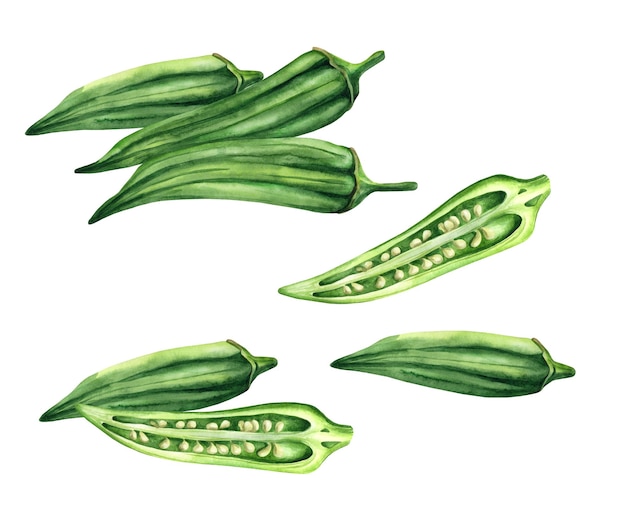This illustration, set against a white background, appears to be a detailed botanical watercolor featuring seven long, slender green pods, possibly okra or peppers, with hints of pale yellow for the seeds. The image is divided into four distinct sections: at the top, three whole pods are laid side by side, showcasing their smooth, green exterior. To the right of this trio, a single pod is sliced open lengthwise, revealing its pithy, seed-filled interior. Below this, on the middle right, lies a short, whole pod, and further down, the bottom right shows another whole pod along with a detailed cross-section of a sliced pod, exposing the pale seeds inside. This meticulous and vivid illustration resembles the kind you might find in a well-crafted cookbook or botanical guide.